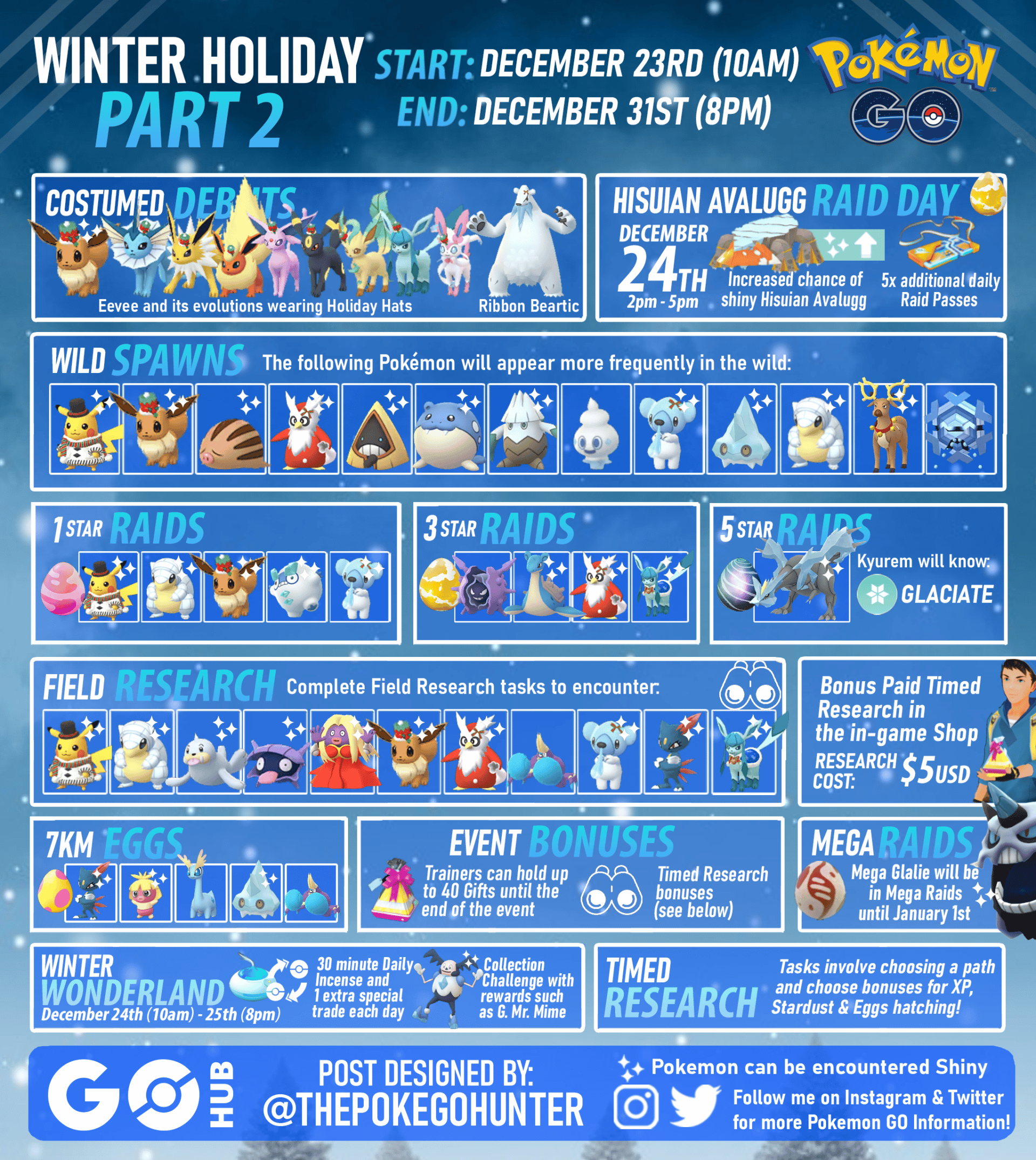The image appears to be a promotional display ad typically seen on websites. The background is a turquoise blue, creating a vibrant and inviting canvas. At the top left corner, "Winter Holiday" is written in bold white font, and directly beneath it, "Part Two" is displayed in a matching turquoise blue font, maintaining the theme. On the upper right-hand corner, the iconic Pokémon logo stands out, featuring "Pokémon" in its signature yellow font with a thin blue outline.

Central to the top of the image, crucial event details are listed: "Start December 23rd, 10 a.m., End December 31st, 8 p.m." Below this information, a captivating collage of numerous Pokémon characters fills the space. These characters are organized into neat rows, each contained within small rectangular sections. The Pokémon vary in color, including shades of gray, orange, brown, and red, adding to the visual appeal. While the individual images of the Pokémon are small and not highly detailed, together they form an engaging and colorful tapestry, drawing fans into the festive event.